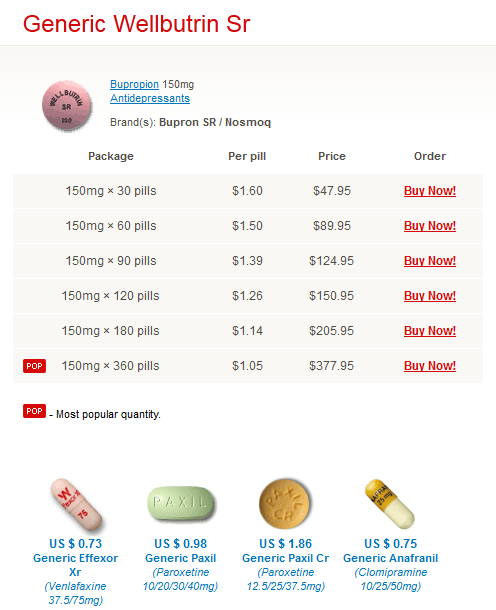This screenshot captures a product page from an online prescription medicine marketplace. The background sports a very light lavender-gray hue. At the top of the page, the product name "Generic Wellbutrin SR" is prominently displayed in red text. Beneath this title, there's a photograph of a round, lavender-colored pill, with the word "Wellbutrin" inscribed in black on its surface. The pill is identified as Bupropion, available in a dosage of 150 milligrams.

Midway down the page, a column on the left-hand side offers options for selecting the quantity of pills, ranging from 150 milligrams times 30 pills to 150 milligrams times 360 pills. At the bottom of the page, additional medication options are displayed, including Paxil, Generic Paxil, and Generic Effexor, suggesting a variety of antidepressant medications available for purchase. The website itself is not identified, as the company name is not visible in the image.